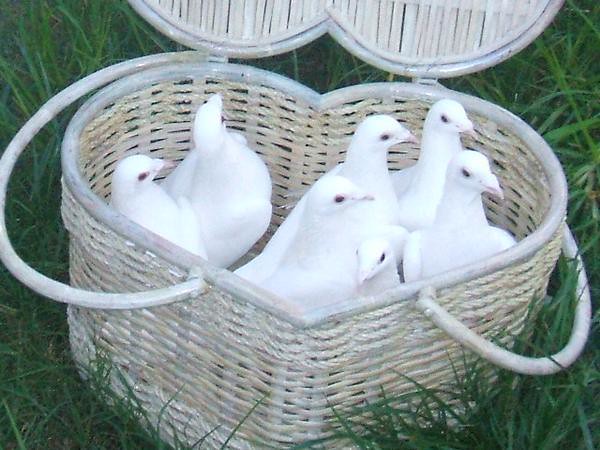The image captures a heart-shaped wicker basket painted white, placed on verdant, vibrant green grass. The basket, adorned with two large handles on either side, has an open lid hinged at its back. Inside the basket, there are seven fluffy white doves, their rounded bodies appearing soft and pristine. The doves' eyes, some of which are visible in a reddish hue, suggest they might be albino. Two doves are nestled in the left corner, while the remaining five are clustered together on the right side. The overall scene is picturesque and serene, showcasing the delicate beauty of the doves against the lush green backdrop.